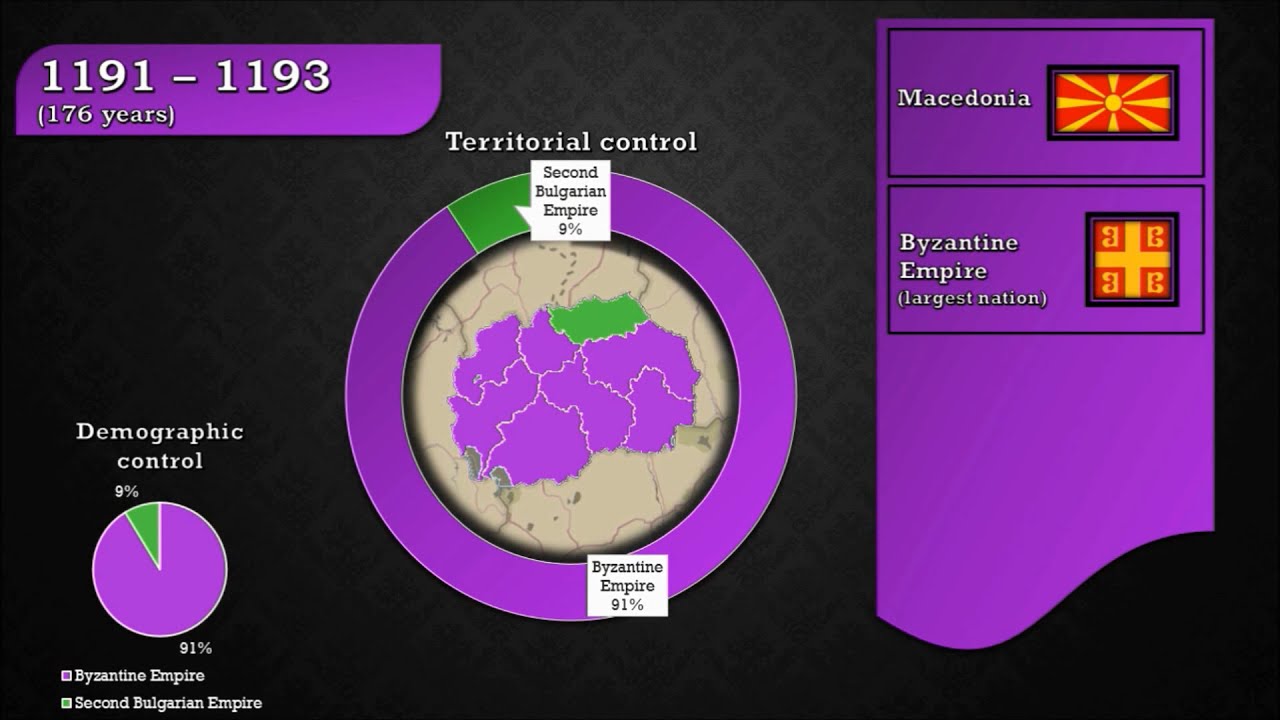This image, appearing to be a screen grab from a historical strategy video game or an informational graphic, showcases a detailed map and several graphs illustrating the territorial dynamics of the Byzantine Empire and the Second Bulgarian Empire between 1191-1193. The background is black, enhancing the vivid colors used for differentiation. The primary feature is a large map divided mainly into purple, representing the Byzantine Empire, with a smaller green section for the Second Bulgarian Empire. 

At the bottom, a pie chart labeled "Demographic Control" visually details the territorial split, with purple covering 91% and green covering 9%. This chart is accompanied by text indicating "Second Bulgarian Empire" for the green segment. Another highlighted element is a purple circle labeled "Territorial Control," prominently featuring a small green slice denoting the Second Bulgarian Empire's 9% share.

In the upper left corner is a purple rectangle with the date range "1191-1193" followed by "176 years" in parentheses. A purple flag accompanied by the text "Macedonia" and the red and yellow sun flag of Macedonia is positioned at the top right, beneath which "Byzantine Empire" is displayed alongside a related yellow and red icon. This highly detailed image serves as both an informative graphic and as an illustrative element in understanding territorial dynamics in a historical context, heavily indicating the predominant control of the Byzantine Empire over this era.